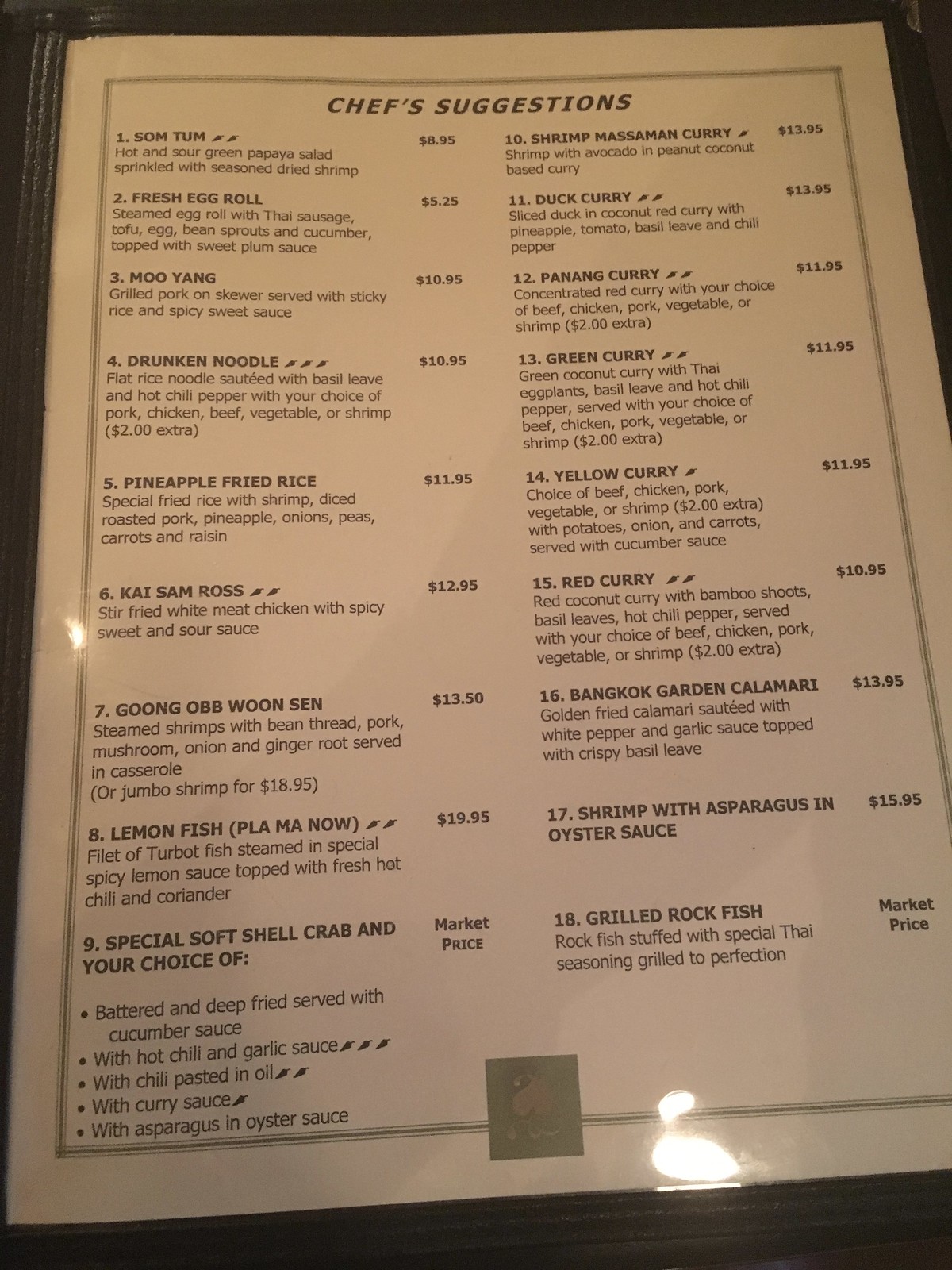The photograph features a slightly dark, color image captured in portrait mode, depicting a page from a restaurant menu. The page is framed with a gray border and shows some glare: a white glare at the bottom and a smaller one on the left-hand side, likely due to lighting reflections.

At the top, the title "CHEF'S SUGGESTIONS" is prominently displayed in bold, all-capital letters. Below the title, the menu is arranged into two columns, listing food items numbered from 1 to 18. Each food item title is highlighted in bold, capital letters, followed by a detailed, non-bold description. The prices for each dish are specified to the right of the item names, varying from $5.25 to $19.95. Additionally, two items are labeled with "market price," indicating variable pricing.

Some of the listed dishes feature illustrations of hot pepper silhouettes next to their names, signifying the spiciness of the item. At the bottom of the menu, a key explains these symbols, providing clarity on the spice levels indicated by the peppers.

Overall, the detailed layout and presentation provide a comprehensive view of the chef's curated selections, including price range and spiciness indicators.